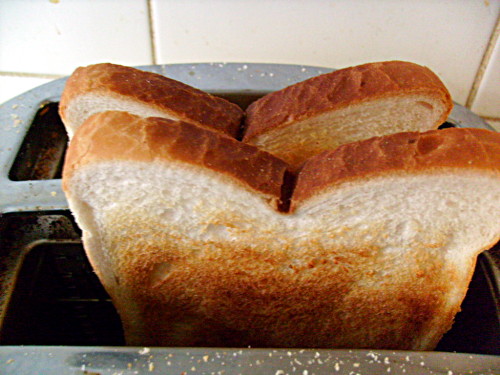This photograph features an extreme close-up of a stainless steel, two-slot vertical toaster, revealing two perfectly toasted slices of white bread with light brown, crisp edges. The focus is on the toaster’s top, capturing the bread in its freshly popped-up position. The metal surface of the toaster is visibly dirty, covered in crumbs and old, burnt residue. The white ceramic tile wall in the background suggests a kitchen setting, adding context to the well-used appliance. The photograph's angle appears to be taken from a slightly elevated position, looking down at the toaster's top, emphasizing the freshly made toast amidst the otherwise grimy surroundings.